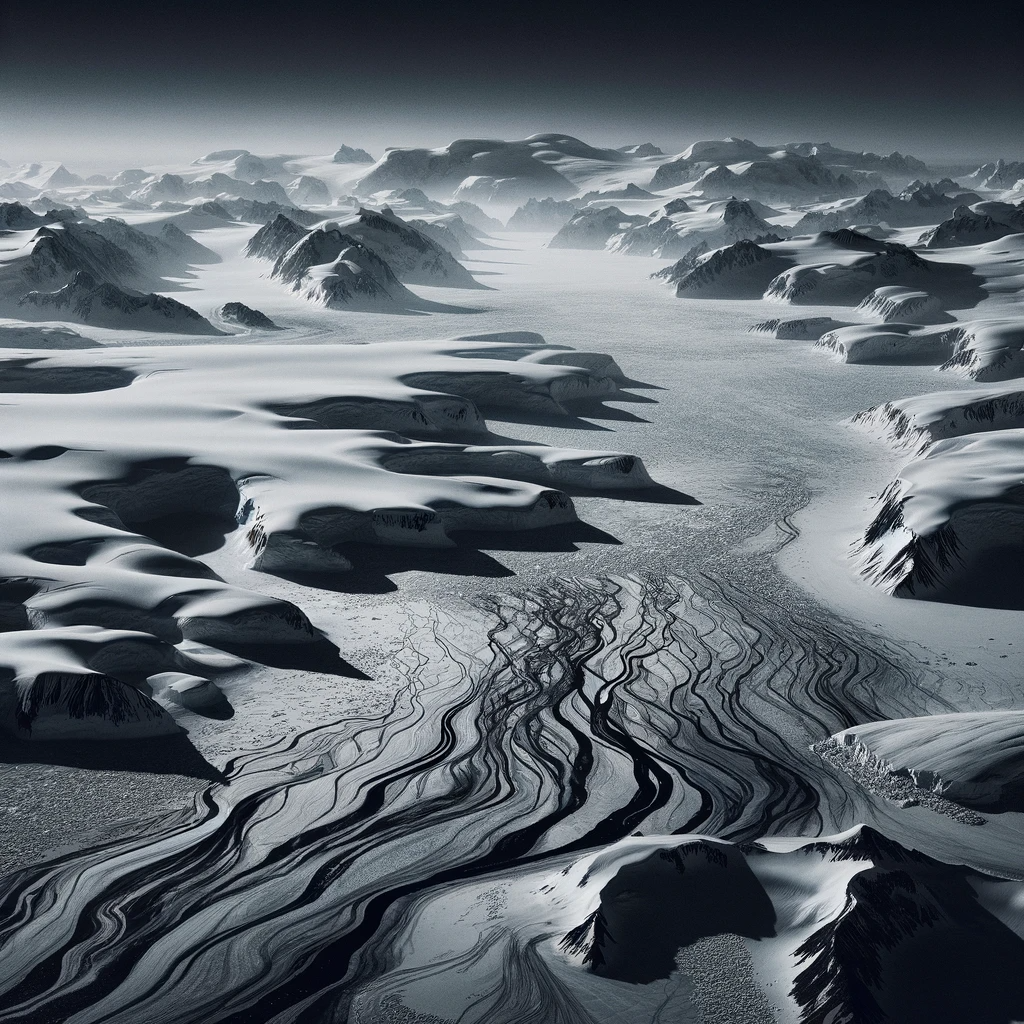In the image, we see a barren, grayscale landscape, whose exact nature is ambiguous—is it a snowy terrain or a sandy desert? The picture is devoid of any trees, people, animals, or vehicles, enhancing its desolate appearance. The top portion of the image features a predominantly black and gray expanse that might represent the sky, though it's unclear whether this suggests nightfall.

The central and lower regions of the image showcase an array of undulating hills and small peaks, with the left and right sides exhibiting steeper formations that could be considered mountains. This rugged terrain varies in texture, with some parts appearing rocky while others are smoother, possibly due to a covering of snow or sand. Notably, toward the center and lower parts of the image, there are intricate, vein-like streaks that converge and intersect, reminiscent of water pathways or ancient river beds, giving an impression of dynamic movement across the terrain.

The overall color scheme includes shades of black, white, and gray, casting a cold, monochromatic ambiance over the scene. Shadows dance across the landscape, especially noticeable in the darker areas, adding depth and complexity to the visual. The lack of textual elements and the empty sky contribute to the mysterious and otherworldly quality of this stark, barren land, which might even belong to another planet.